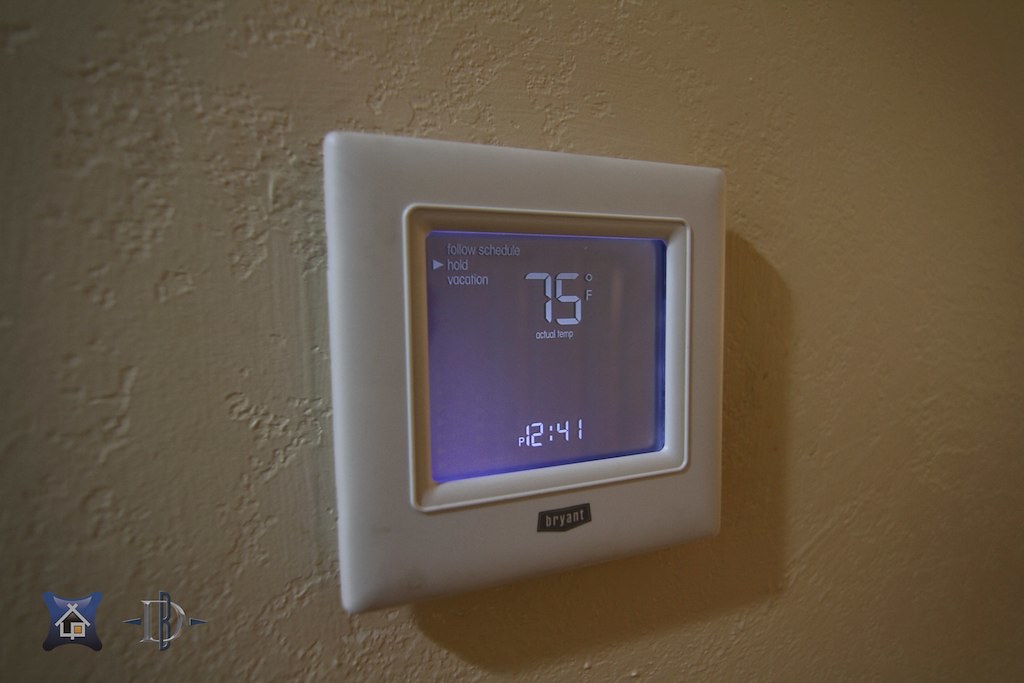This photograph captures a detailed interior scene. On the left side, a whimsical square frame features a stick-figure house, adding a touch of playful artistry. Adjacent to this frame, two prominent letters, a "D" and a "B", are mounted on a white wall, which is textured with decorative chips. Centrally placed on the wall is an electric thermostat encased in a thick white plastic frame. The thermostat’s display screen, which appears blue-green, reads "Follow Schedule" at the top with "Hold" and a pointing arrow below it. The word "Vacation" is noted further down, and the current temperature is prominently displayed as "75°F, Actual Temp." The bottom of the screen shows "P12.41." The brand name "BRYANT" is printed on the plastic casing of the thermostat, standing out against its gray background. This intricate setup combines both functional and aesthetic elements harmoniously in the space.